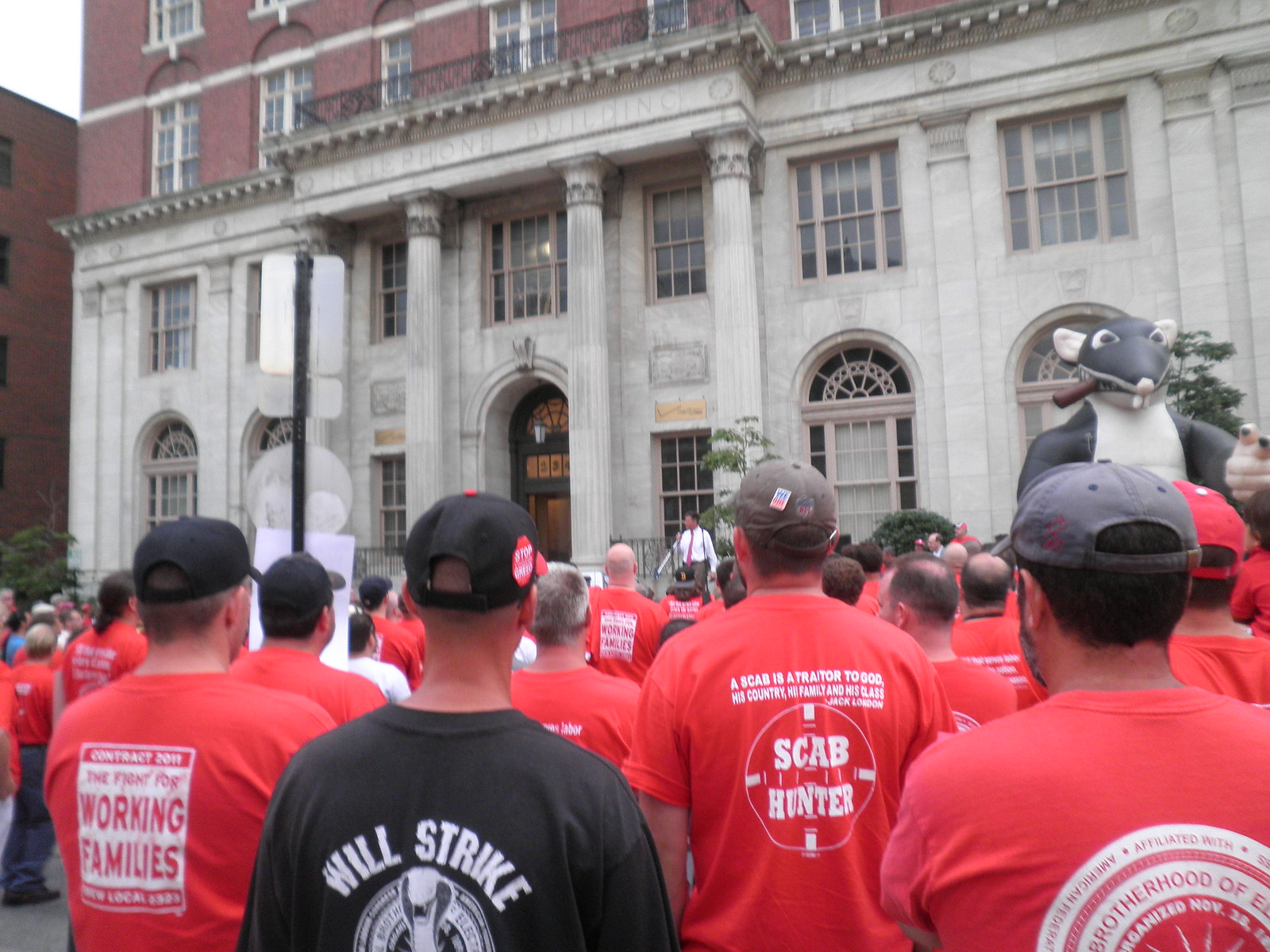The image captures a dynamic protest or rally in front of an imposing building, which displays prominent British architecture characteristics. The lower floors of the building feature light gray stone masonry with vintage patterned doors, large windows, and grand pillars. Above, the upper floors are made of brick, adorned with large windows and balconies, accented by a pink exterior paint.

The event is taking place during the daytime, as evidenced by the clear sky. A man, small in the image but centrally positioned, stands at a microphone. He is dressed in a white long-sleeved shirt, a pink tie, and brown pants, with dark hair, appearing to address the crowd.

In the foreground, a large crowd, probably over 100 adults, predominantly male, face away from the camera, all wearing matching red t-shirts, except for one individual in black. The red t-shirts feature various slogans such as "Contract 2 in 2011, the fight for working families" and "a scab is a traitor to God, his country, his family and his class, Jack London," with some displaying a "Scab Hunter" logo. The man in black wears a shirt that reads "Will Strike," emblazoned with a snake graphic.

Amidst the crowd, partially facing towards the camera, stands a striking inflatable rat, about 12 feet tall, puffing a cigar, accentuating the protest's fervent atmosphere. The building behind them is identified as the "Telephone Building," evidenced by the writing above its grand columns, contributing to the setting’s historical and architectural gravitas.